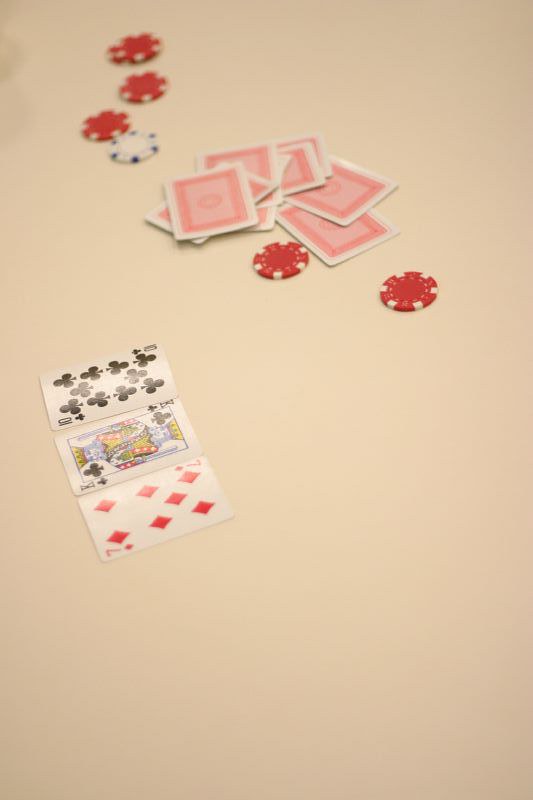This vertically oriented photograph captures a poker scene set against a beige background. Central to the composition, there are three playing cards neatly arranged at a slight leftward angle: the Seven of Diamonds, the King of Clubs, and the Ten of Clubs. Just above and to the right of these cards lies a neatly stacked semicircular pile of cards, showcasing red backs adorned with a circular pattern in the center. Each card also features a darker red border encircled by a thin white edge. 

In the upper left section of the photograph, four poker chips are visible. Three of these are red with distinctive wedge-shaped white accents forming a dotted pattern around the edges, while the fourth chip, positioned at the bottom, is white with similar blue wedge-like shapes. Directly beneath the arch of playing cards rests an additional red poker chip with white accents, and another red chip with identical white markings is located slightly to the right and below it. The photograph meticulously captures the arrangement and details of the cards and poker chips, reflecting an engaging moment of a poker game in progress.